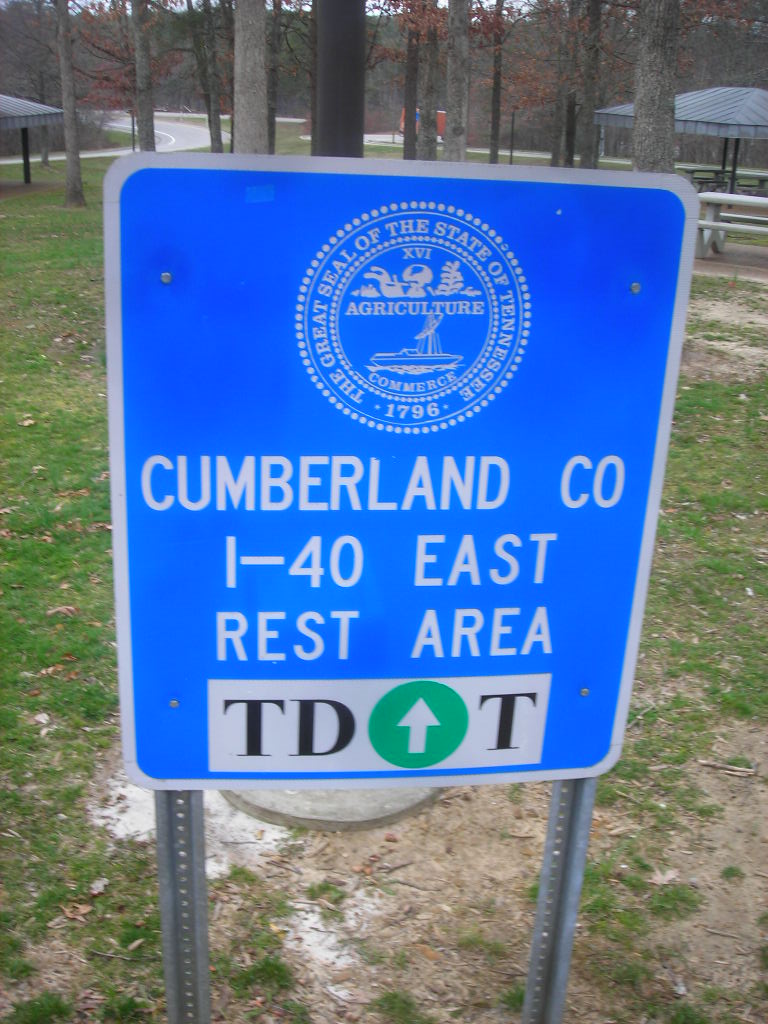This outdoor daytime photograph features a prominently blue sign with a silver outline, mounted on two steel vertical brackets. The sign displays the Great Seal of the State of Tennessee, labeled with "Agriculture" and "Commerce" and dated "1796" in a circular design at the top. Below the seal, in white capital letters, the sign reads: "Cumberland Co." followed by "I-40 East," then "Rest Area." Beneath this, a white rectangular section bears the black letters "TD," alongside a green circle containing an upward-pointing white arrow and a black "T." The backdrop reveals a park-like setting with grass, sparse areas, and about 10 to 12 tree trunks visible far in the upper portion. To the upper right of the image, a pavilion is noticeable, while the upper left shows part of a curved road extending away. Concrete picnic tables are dispersed among the trees, suggesting a rest area ambiance, possibly in the fall due to the sparse foliage.